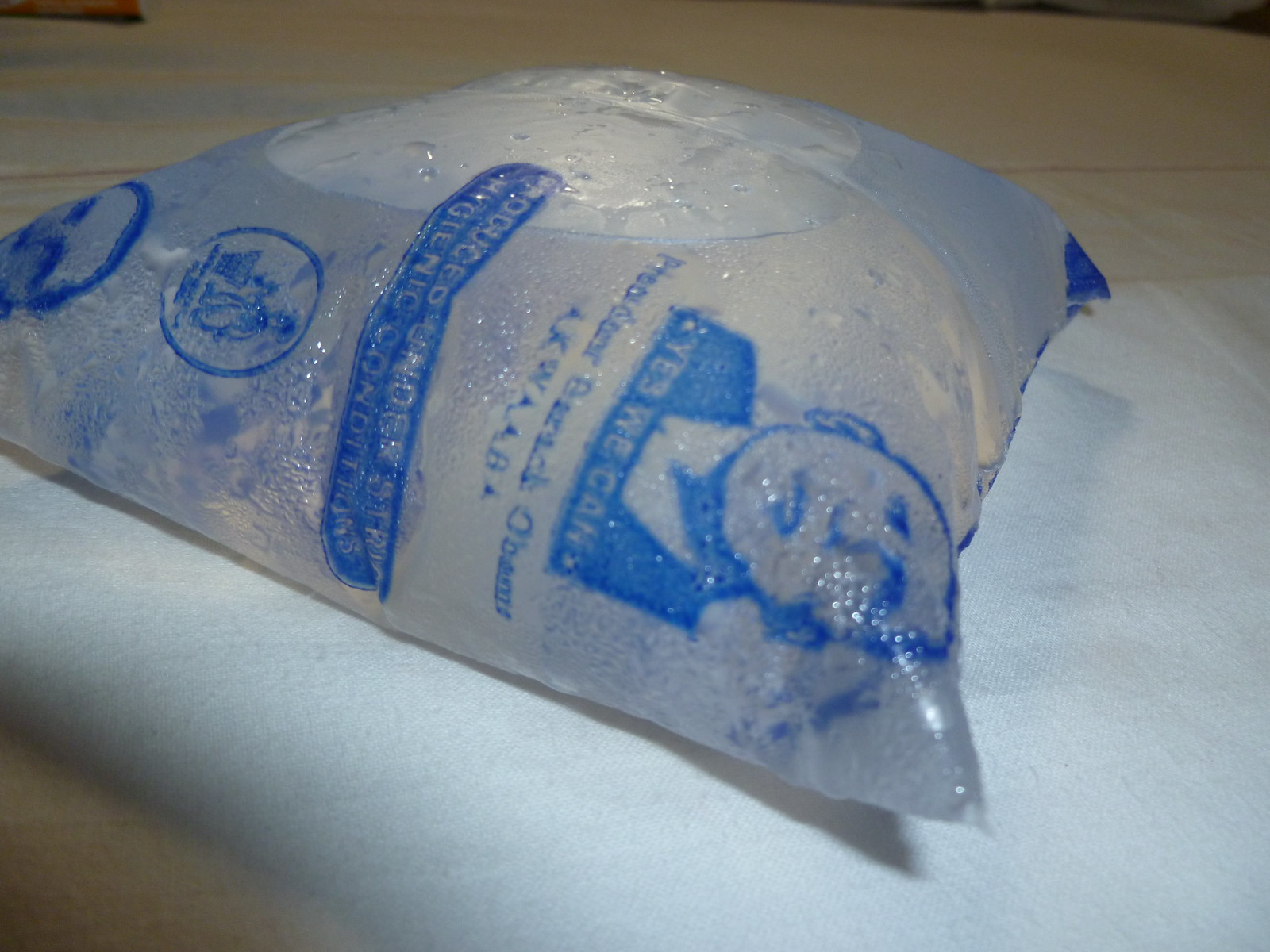The image depicts a melted ice pack resting on a hybrid white and blue blanket, possibly on a concrete surface given a visible line suggesting a driveway. The ice pack is now just water with condensation on the exterior. The packaging features prominent, royal blue text and images, including the phrase "Yes We Can," "A-K-W-A-A-B-A," and mentions President Barack Obama, with a somewhat distorted cartoon-like face of him due to the melted state of the bag. There are additional blue graphics, including a rectangle of text and a circle indicating proper disposal instructions, advising against throwing the bag in the trash.